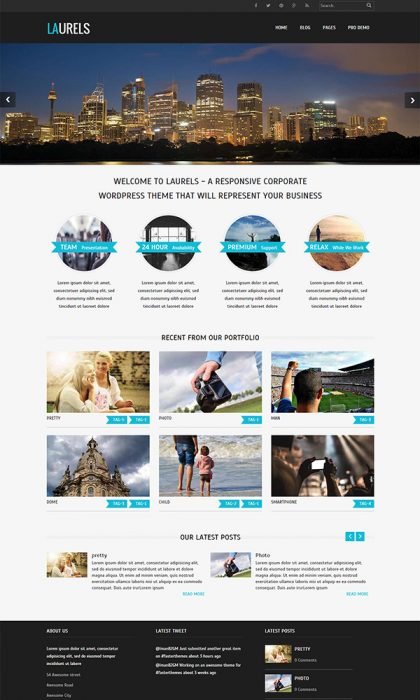This photograph captures a mobile phone screen displaying the homepage of the "Laurels" corporate WordPress theme. The title "Laurels" is prominently featured, with "L-A" highlighted in blue and "U-R-E-L-S" in white. The background showcases a bustling, illuminated cityscape at dusk, featuring towering skyscrapers with their lights aglow. At the top of the screen, navigation links such as "Home" and other sections are visible.

Centered on the page is a welcoming message: "Welcome to Laurels, a responsive corporate WordPress theme that will represent your business." Below this, three or four circular icons describe features such as "Team Recognition," "Team Presentation," "24-hour Premium Support," and "Relax."

Scrolling further down, the section titled "Recent from Our Portfolio" displays six images arranged in two rows of three, showcasing the company's latest projects. Beneath this is another section labeled "Our Latest Post," featuring two articles: "Pretty" and "Photo." The "Pretty" post includes an image of two women sitting next to each other, one gazing at the other. The "Photo" post features an image focused on a person holding a camera, with the scene's attention drawn solely to the camera.